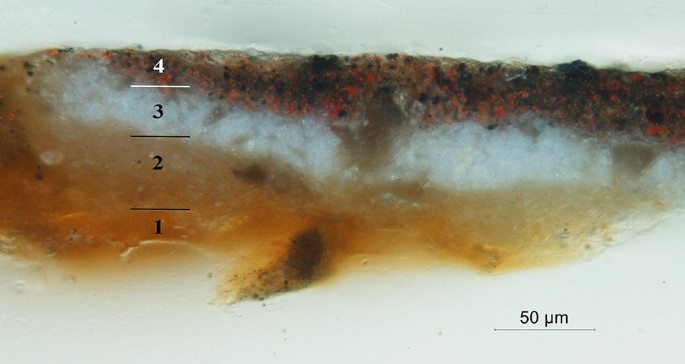The image is an abstract depiction that appears as a long rectangular horizontal frame divided into four distinct layers, each numbered sequentially from 1 to 4. The bottom layer (1) is predominantly off-white, transitioning to an orangish-brown color about a third of the way up. The second layer (2) above it showcases a lighter brown gradient. The third layer (3) is characterized by a cloudy white abstract line. The topmost layer (4) features a darker palette of black, brown, and red hues, speckled with some orange spots.

Adjacent to these layers, on the bottom right corner, sits a measurement scale labeled "50 UM," indicating that the image is likely portraying a microscopic view, possibly of sediment or microbial samples. The overall image's abstract nature and ornate details make it challenging to identify precisely but evoke impressions of geological or biological material. The composition and the numbered scale suggest a scientific context, as if illustrating layers within a beaker or a geological sample viewed under a microscope.